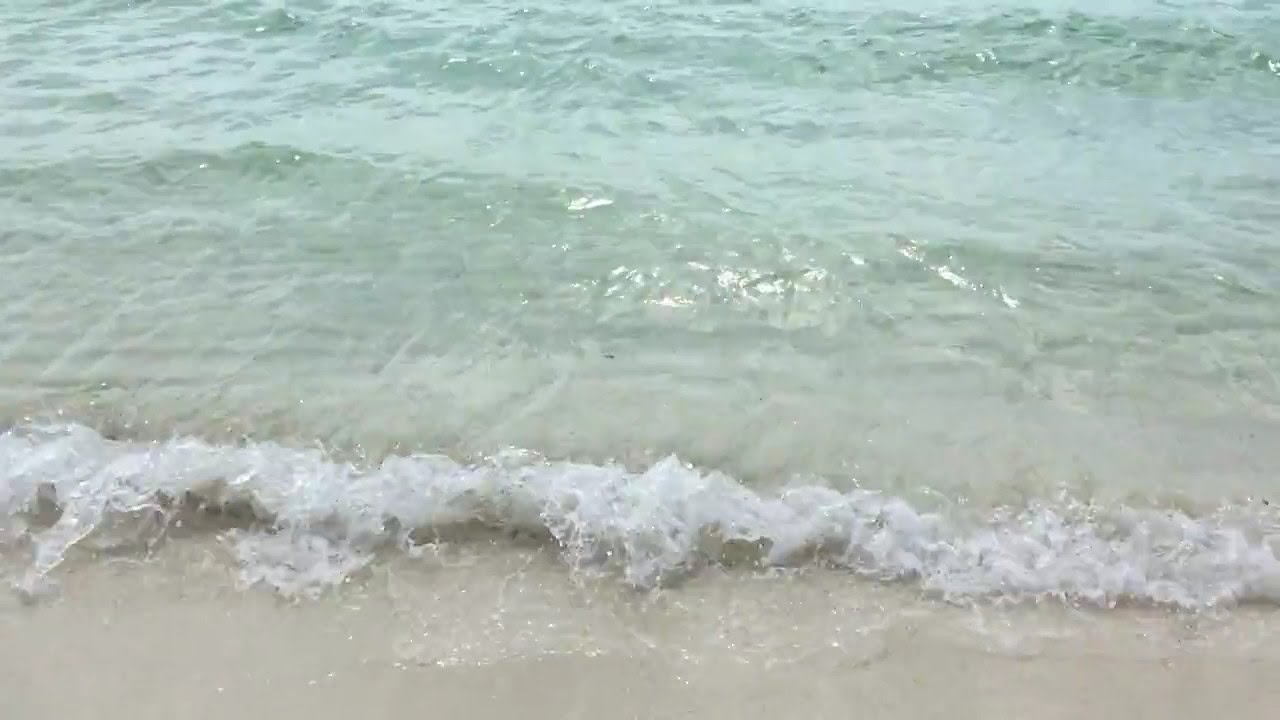The image captures a tranquil beach shoreline with an emphasis on the pristine, light greenish-blue water that dominates the scene. At the bottom edge of the photo, a slender strip of smooth, fine, light-colored sand marks the shore. This is where gentle waves break, creating a frothy, white edge as they crash onto the sand. The clear water reveals the seabed underneath, highlighting its transparency. The overall setting appears to be outdoors, during daylight, with no people, animals, or text present, solely focusing on the natural beauty of the beach and the serene interaction between the sand and the water. The colors predominantly include light green, white, and tan, adding to the peaceful and unspoiled ambiance of the scene.